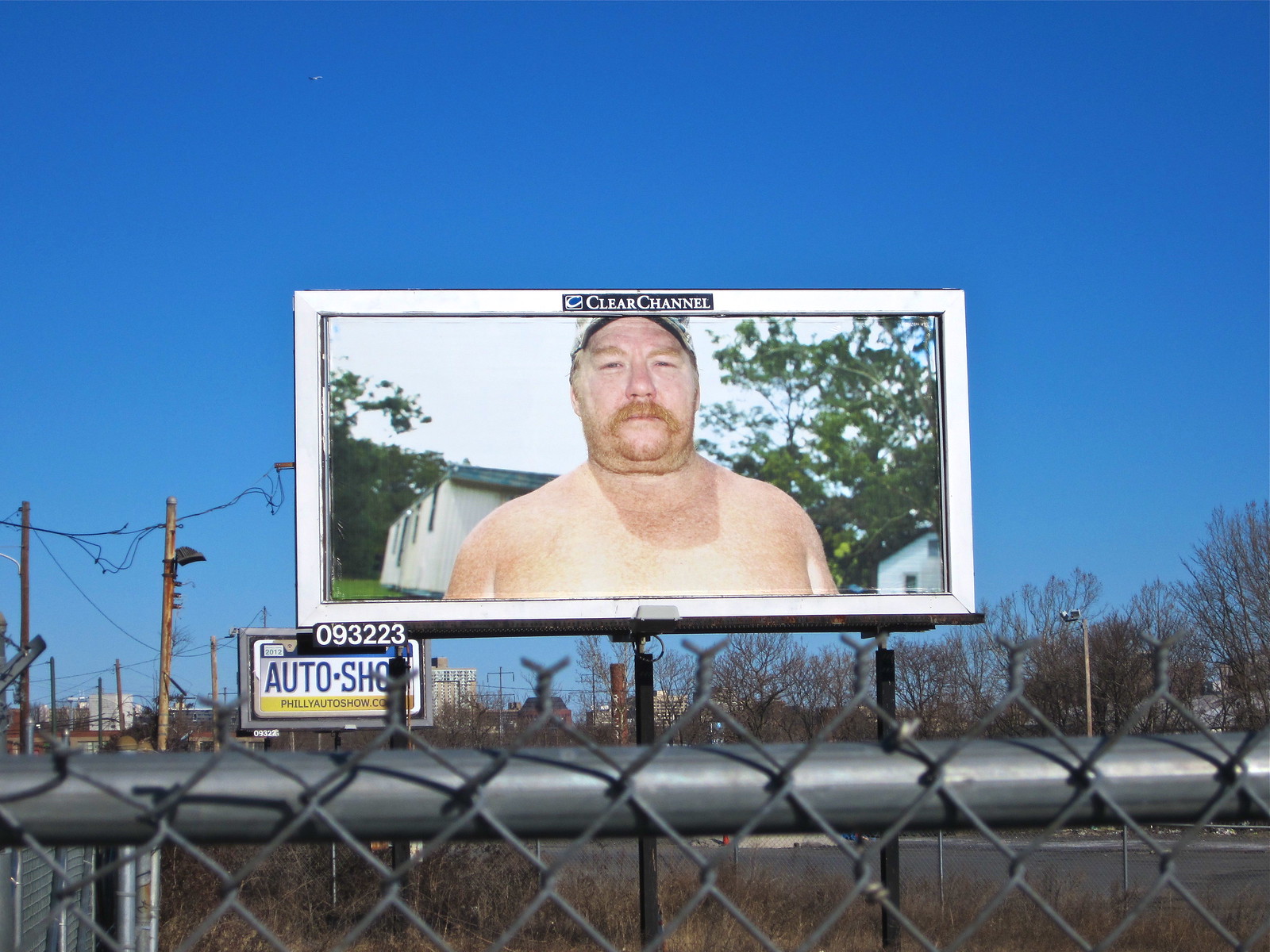The image is a slightly horizontally rectangular photograph capturing a stark, autumn landscape. Dominating the lower part of the frame is the upper section of a chain link fence, including its top horizontal bar. This fence serves as a barrier between the viewer and the scene beyond, where leafless, barren trees stretch upward, indicating the fall season. Rising above the trees, the background transitions into a vast expanse of deep blue sky, completely devoid of clouds, lending an almost surreal, uninterrupted backdrop to the image.

At the heart of the composition, behind the chain link fence, stands a large billboard with a prominent white border. On the top border, centered, the words "Clear Channel" are clearly visible, identifying the billboard's managing company. The advertisement features a striking visual: a shirtless, portly man shown from the chest up. His most distinguishing feature is a full, vibrant red mustache that cascades down the sides of his face, adding a touch of personality and intrigue to the scene.